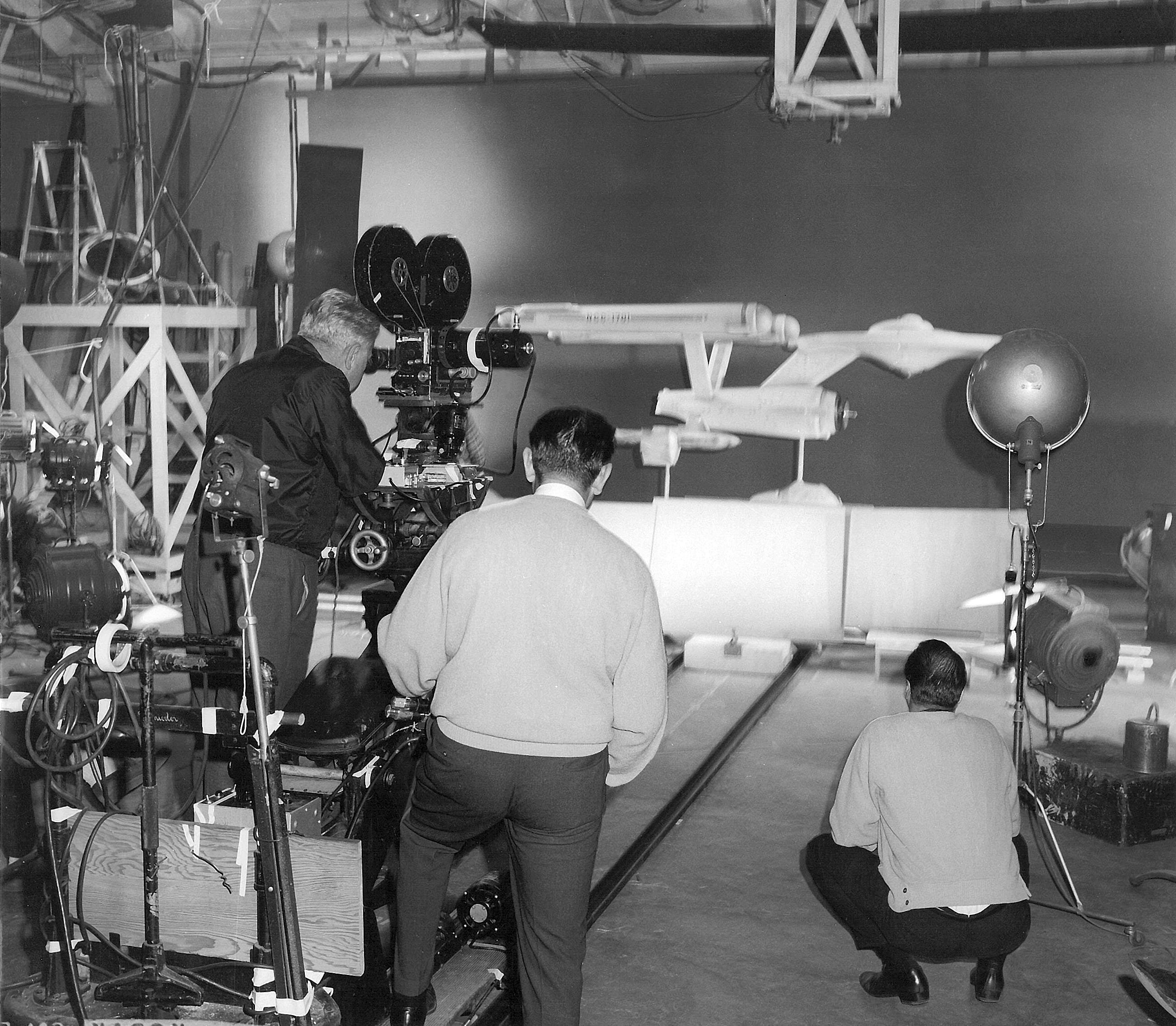This black-and-white photograph, likely taken in the 1940s or 1950s, captures a film set featuring a large model of a spaceship that resembles designs from the Star Trek series. The focus of the image is the spaceship, which rests on a wide rectangular platform. In the foreground, three men are seen from behind, each engaged with different aspects of the production. On the left, an older man with silvery white hair operates a large film camera mounted on tracks, aimed at the spaceship. He wears dark pants and a dark long-sleeve shirt. Beside him stands a man with dark hair, dressed in dark pants and a light-colored sweater, who appears to be involved with the cameras or other filming equipment. To the right, another man with dark hair is squatting near a light fixture, dressed similarly in dark pants and a light-colored sweater, seemingly in charge of lighting. The left side of the photograph features wooden scaffolding and wiring, along with various set props and items, adding to the vintage atmosphere of the scene.